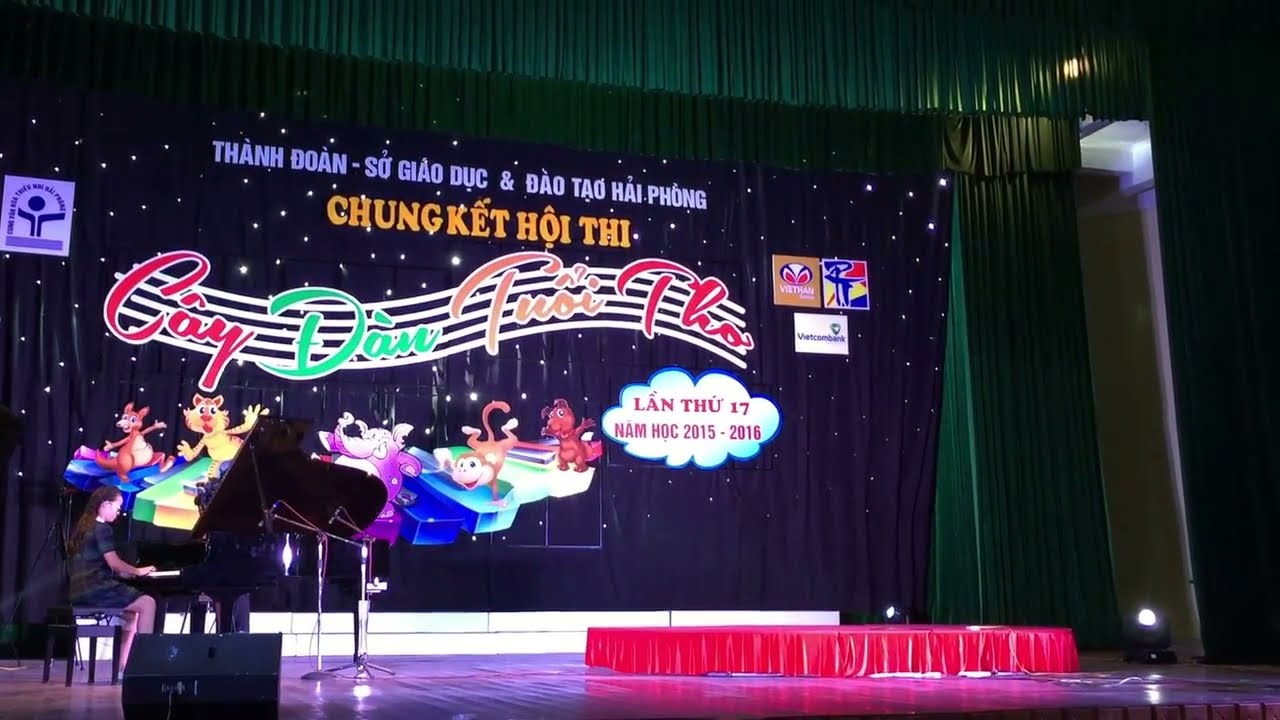This full-color photograph, taken indoors from the audience's perspective, captures a stage set for a musical performance, likely a school talent show in Vietnam. Dominating the left side is a young girl with long dark hair, dressed in a striped dark dress, seated on a stool and playing a piano. The stage is framed by green and purple curtains, with a blue poster hanging at the back. The poster features multiple layers of text and images. At the top, purple Vietnamese text reads "Thanh Doan So Giau Duc" and "Dao Thao Hai Phong." Below, more Vietnamese words appear in lavender and gold fonts. A series of wavy white lines resembling musical staffs run across the poster, adorned with additional Vietnamese words in red, green, and orange italics. Below the text are cartoon animals, including one playing a piano, adding a playful touch to the scene. In the center of the stage, covered with a red cloth, stands a separate podium. The overall composition suggests an event meant to showcase children's musical talents.